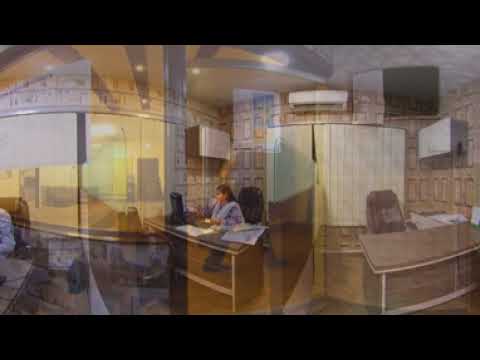This photograph depicts the interior of an office room as seen through a glass window, evident from various reflections on the glass surface. At the center of the image, a woman is seated on a black chair behind a desk, working on a desktop computer. The desk has scattered papers on it. Behind the woman, attached to the wall, there is a cabinet and an air conditioner unit mounted above cream-colored curtains that cover a window. The ceiling is designer with integrated lights, and a door is visible on the far left. To her left, there is a partition, separating her space from another smaller cabin that contains an empty desk with a chair, surrounded by files and papers, and another wall cabinet. The image has a curved distortion at the top and bottom, accentuated by horizontal black strips, and appears blurry and shadowed, possibly from an overlaid or superimposed image, casting an unclear and reflective quality.